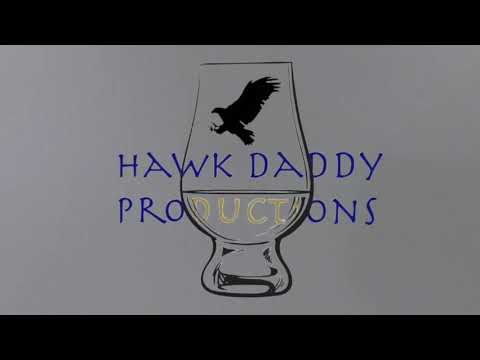This image is a stylized, logo-like graphic set against a large gray rectangular background. At its center, the words "Hawk Daddy Productions" are prominently displayed. The words "Hawk" and "Daddy" are in a vivid blue color, while the word "Productions" is mostly blue with the letters D-U-C-T highlighted in a golden yellow color. Overlaying these words is a transparent, 3D-rendered snifter glass, allowing portions of the text to be visible through its transparent form. Positioned inside the upper part of the glass is a silhouette of a hawk, rendered entirely in black. The image is framed at the top and bottom by horizontal black banners, lending a centered and framed appearance to the composition. The overall design evokes the feel of a professional logo, possibly for an entity named "Hawk Daddy Productions."